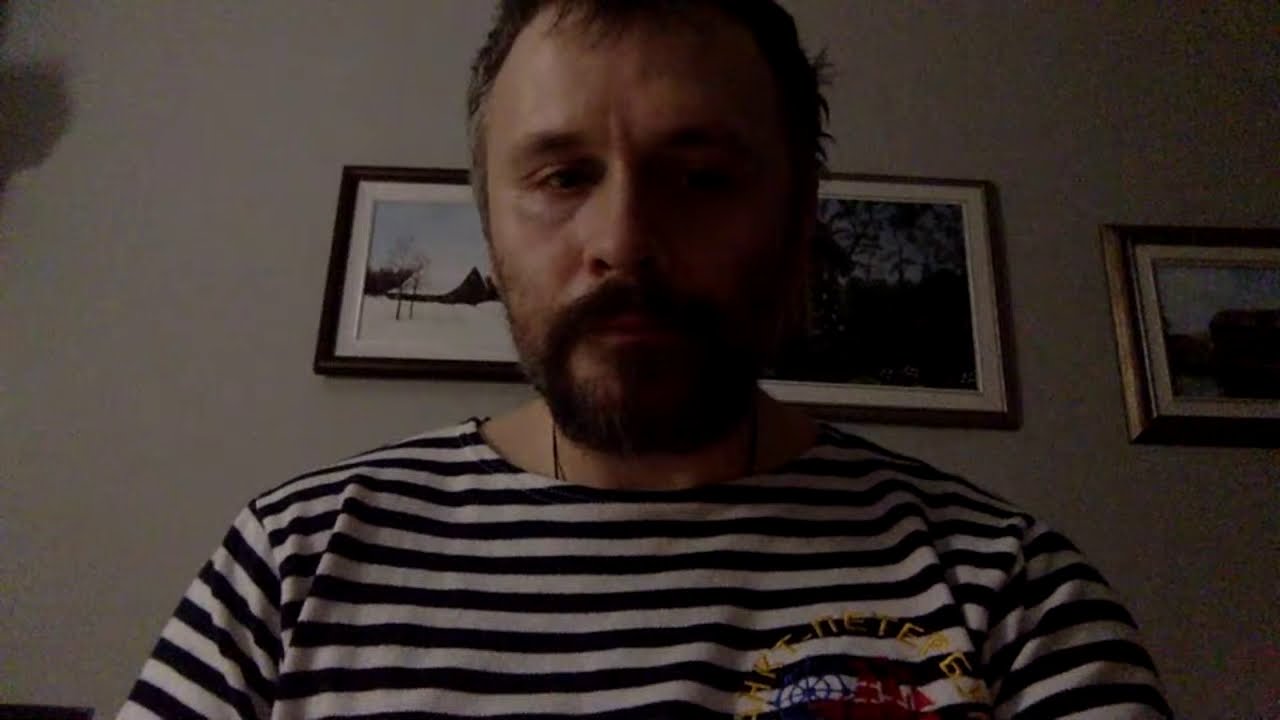The image captures a close-up of a middle-aged man sitting in a dimly lit room, which creates a gradient effect from left to right, transitioning from lighter to darker and becoming grainy in the darker areas. He has short gray and brown hair, a short brown beard, and white skin. The man is wearing a white and black striped shirt, reminiscent of a sailor design, with a barely visible circular logo or crest on the left shoulder, and he appears to be wearing a thin necklace underneath. The framing shows him from the chest up, and he is slightly elevated above the camera, looking off to the side with a furrowed brow, giving an impression that he is in a bad mood. The wall behind him is neutral in color and adorned with two or three small framed pictures, one of which seems to depict a snowy cabin.